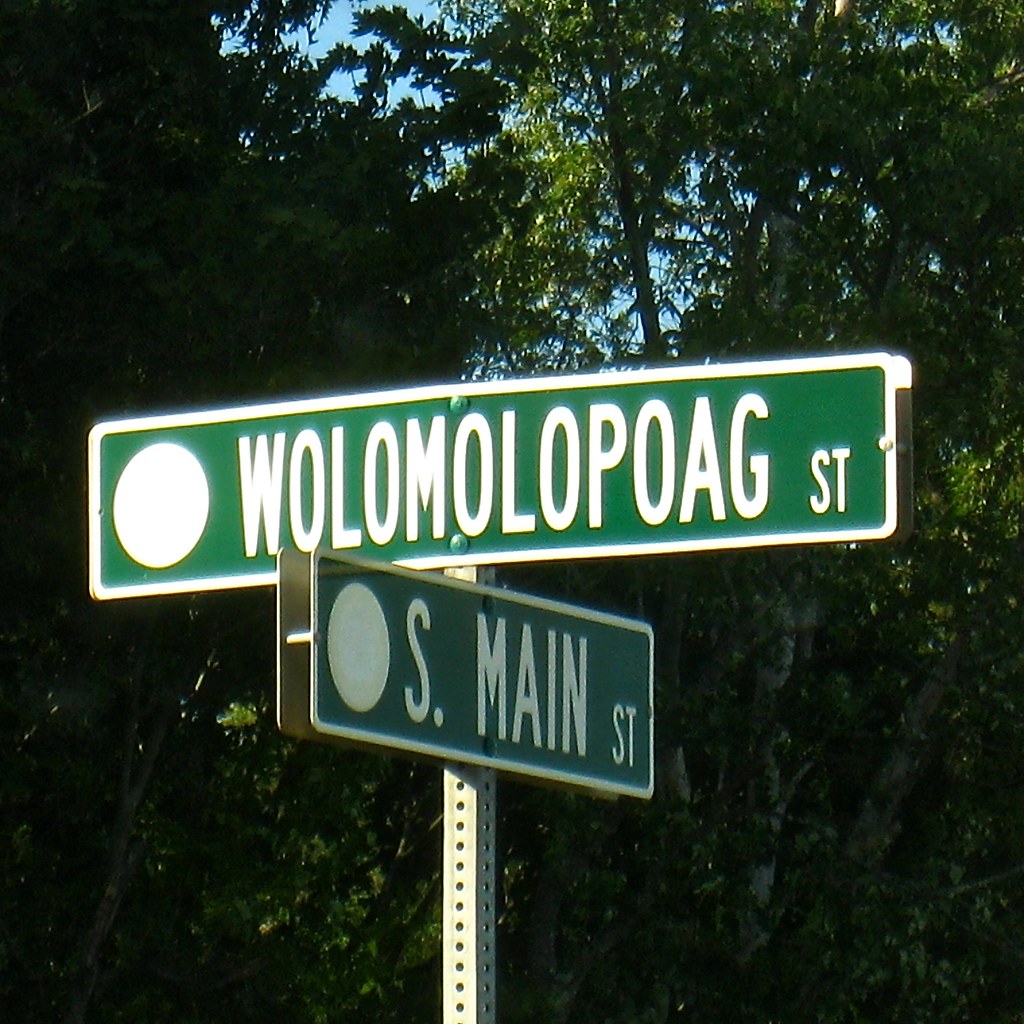The image features a close-up view of two green street signs, each framed with a white border and featuring a solid white circle on the left side. The top sign reads "Wolomolopoag Street" in white text, while the sign below it reads "S. Main Street." Both signs are attached to a rectangular, silver steel pole with numerous vertically aligned holes. The signs are oriented at different angles; one is horizontal, and the other is slightly tilted. In the background, dense green foliage from trees and patches of bright blue sky are visible, suggesting a sunny day with ample natural light illuminating the scene.